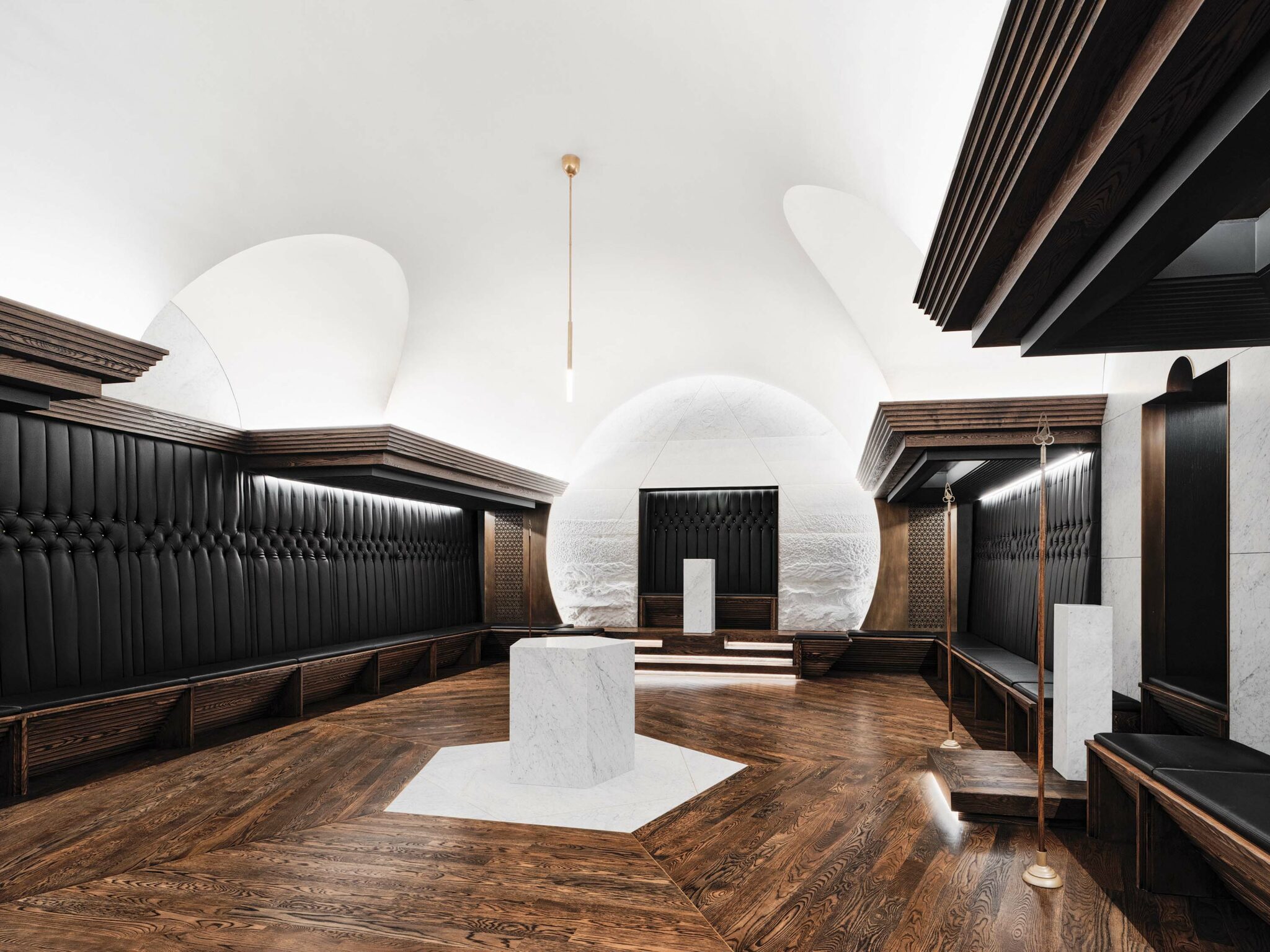This image showcases a vibrant, ultra-modern lobby or room that blurs the line between reality and digital construction. The space features a harmonious blend of luxurious materials—wood, marble, and leather. The room’s focal point is a white, multi-sided marble pedestal, either hexagonal or pentagonal, set on a wooden floor. Surrounding this central piece, the elegant floor transitions seamlessly from marble to dark brown wood, adding warmth to the interior. 

The ceiling above is pristine white, adorned with curved lines and cutouts that frame hidden light fixtures, adding an element of sophistication. One curved section even features a thin, hanging gold pendant plate that enhances the room's opulent feel. Toward the back of the room, a circular structure with undulating white and gray patterns houses a marble podium with a black leather background, and steps leading up to it – likely indicating an entrance or exit. 

The walls are lined with wooden benches featuring black leather cushions and backs, continuing the use of high-quality materials. The leather extends up the walls in a tufted pattern, capped with dark brown wooden edging. The symmetry, choice of materials, and sophisticated design elements make this space both striking and contemplative.